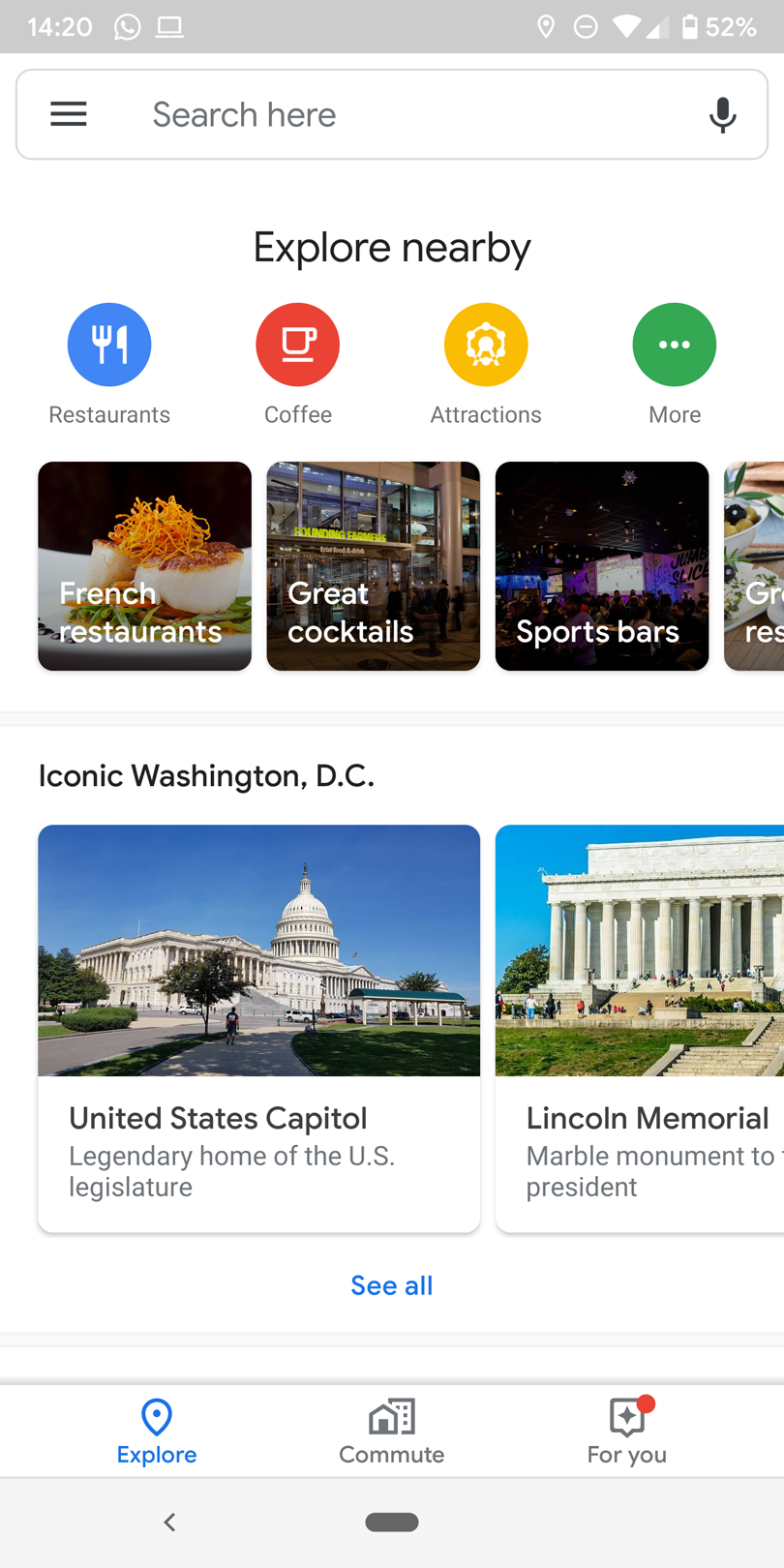The image, displayed on a smartphone, provides a detailed snapshot of a local exploration app interface. The phone's screen shows a battery life of 52% and a strong connection, with the time reading 14:20. The top of the screen features an empty search bar with the prompt "Search here" and a microphone icon, all rendered in gray and white tones. Beneath the search bar, the text "Explore nearby" appears in black.

A series of categorized options follows, each represented with distinct icons and colored circles: "Restaurants," illustrated by a fork and knife in a blue circle; "Coffee," depicted by a coffee cup in a red circle; "Attractions," shown with an attraction icon in a gold circle; and "More," indicated by three dots in a green circle.

Below these categories are photographic thumbnails showcasing actual French restaurants, delicious dishes, and vibrant cocktails. The images also highlight a sports bar, but the fourth image is partially cut off and not visible in its entirety. The locale is identified as Washington, D.C., with accompanying photographs of the United States Capitol and the Lincoln Memorial, complete with brief descriptions. A clickable "See all" option in blue text invites further exploration.

At the bottom of the screen, navigation options are displayed: "Explore" in blue, "Commute" in black and white, and "For you" in black and white with a red dot above it, indicating notifications or new content.